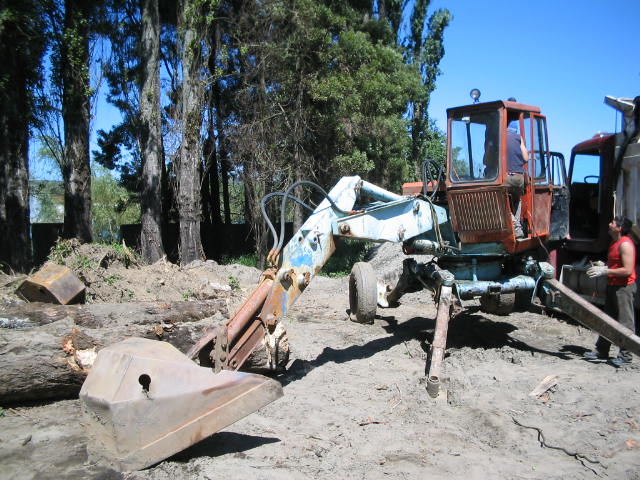The photograph depicts a bustling construction site set against a backdrop of lush greenery and a bright blue sky. In the foreground, the ground is uneven and torn up, indicative of recent heavy work, with fallen tree trunks scattered on the left side. Dominating the right side of the image is a weathered backhoe, primarily orangish with hints of faded blue, suggesting an older, well-used machine. The backhoe's arm, ending in a dusty gray spade or shovel, rests on the ground, and inside the red-caged cabin, a person stands with their back to the camera. Adjacent to the backhoe is a large truck with its door open, partially visible. A man wearing a red tank top and dusty gray pants stands on the right edge of the photograph, looking up and seemingly conversing with the operator inside the backhoe's cabin. The entire scene is framed by a stand of upright trees with green leaves, enhancing the natural beauty of the site despite the construction activity.